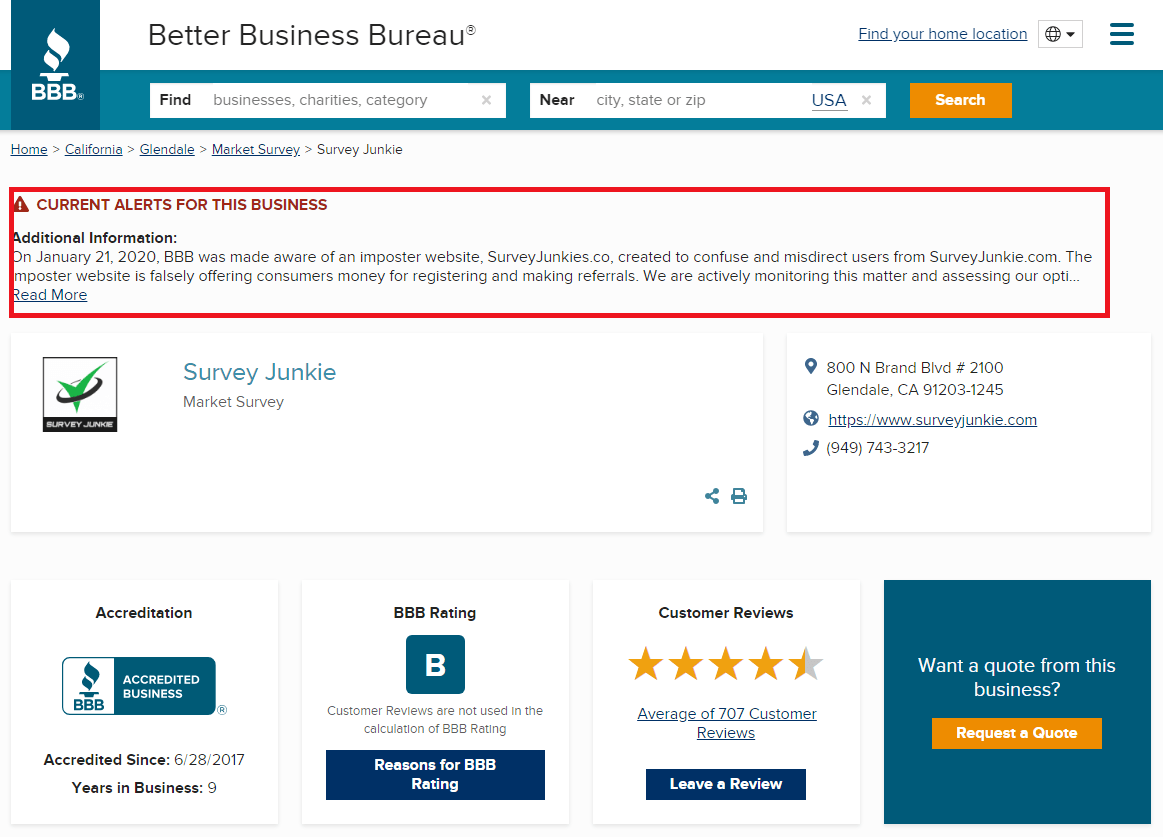**Detailed Caption:**

This is a screenshot of a web page from the Better Business Bureau (BBB). At the top of the page, against a white background, the text "Better Business Bureau TM" is prominently displayed in black font. To the right of this text, there is an underlined blue font link that reads "Find your home location." In the center, a small black-outlined rectangle houses a globe icon, accompanied by a downward-pointing arrow indicating a drop-down menu. To the right of this, three blue horizontal lines likely represent a menu icon.

Below the main header, the BBB's logo is featured: a torch with three white "B" letters stacked on top of each other, set against a blue background. The website's search functionality follows, consisting of two fields. The first field is for finding "businesses, charities, category," and the second for specifying the "near, city, state, or zip" location. An orange "Search" button with white font appears next to these fields.

Further down, there are navigation links including "Home," "California," "Glendale," "Market Survey," and "Survey Junkie." Below this, framed in a red outline, is a warning message. The alert states that on January 21, 2020, the BBB was informed about an imposter website, surveyjunkies.com, which was created to confuse and misdirect users from the legitimate site, surveyjunkie.com.